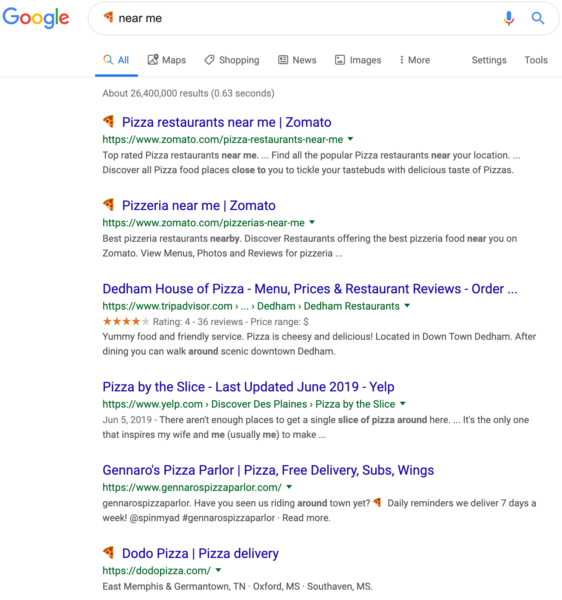The image features a search engine interface with a white background. At the top, there is a Google search bar displaying the query "pizza restaurants near me," which includes a microphone icon and a magnifying glass icon for voice search and standard search input, respectively. Below the search bar, the options "All" (highlighted with a blue underline), "Maps," "Shopping," "News," "Images," "More," and "Settings & Tools" are visible.

The search results include:
1. A Zomato link for "Pizzeria near me," mentioning the establishment "Dead Ham House of Pizza," along with menu prices and restaurant reviews, followed by an order prompt marked by ellipses.
2. A Yelp entry for "Pizza by the slice," last updated in June 2019, featuring "Genero's Pizza" offering pizza, free delivery, subs, and wings.
3. A website link for "Dodo Pizza" with the URL "https://dodopizza.com/," indicated by a down arrow.

The regional locations covered in the search results include East Memphis and Germantown, TN; Oxford, MS; and Southaven, MS.